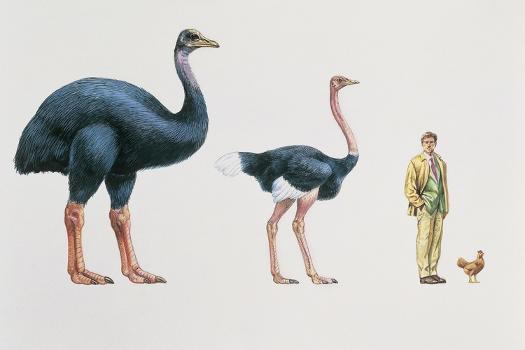The colored pencil drawing illustrates a comparative size and detail study of an extinct, primitive ostrich-like bird, a modern-day ostrich, a man, and a chicken. On the far left, the extinct bird stands impressively large and imposing, covered in thick, dark feathers from its head to its stout tail. Unlike modern birds, it has no visible wings, a robust neck also clad in feathers, and hefty legs. Centered in the image is a modern ostrich, noticeably smaller than its ancient counterpart. This ostrich features black body feathers with white-tipped wings and a white tail. Its long, skinny neck and head are pink and fleshy, with smooth legs lacking any feathering. To the right of the modern ostrich stands a man dressed in a yellow suit with a green vest. He is shorter than both birds, adding a sense of scale to the image. Lastly, positioned to the right of the man is a small, round chicken or rooster, which completes the size comparison and highlights the evolutionary spectrum of these birds.